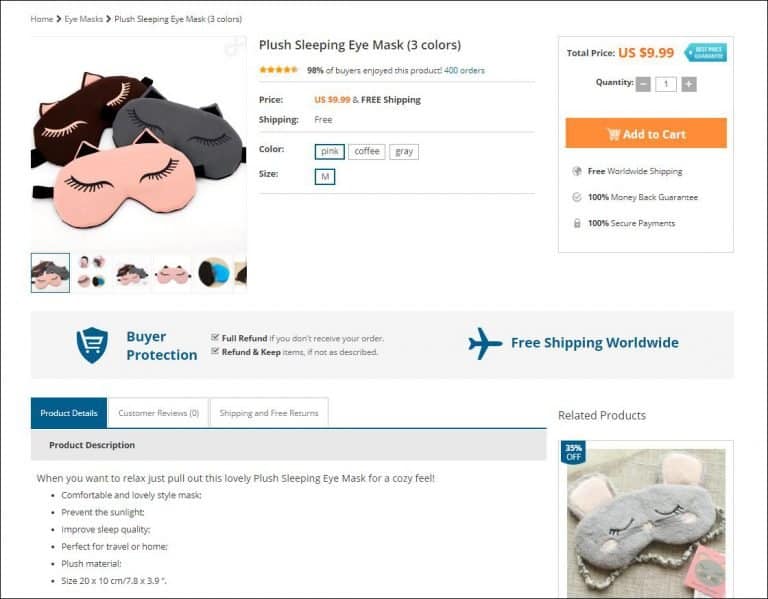This image showcases a collection of plush sleeping eye masks available in three colors: pink, gray, and brown. Each mask is adorned with adorable cat ears at the top, enhancing their playful and cute appearance. The pink mask mimics a fair skin tone with delicately drawn, closed eyes lined with eyelashes, creating a serene sleeping face. The gray mask features a neutral face with cat ears, adding to its charm. Similarly, the brown mask also has the distinctive cat ears, maintaining a consistent theme across all masks.

The masks are promoted as a medium size and are described as perfect for both travel and home use. Made from plush material, they are designed to block sunlight effectively, thereby improving sleep quality. The product description emphasizes comfort and style, highlighting the masks' cozy feel. Additionally, the promotion mentions a 35% discount, making these lovely sleep aids even more attractive.